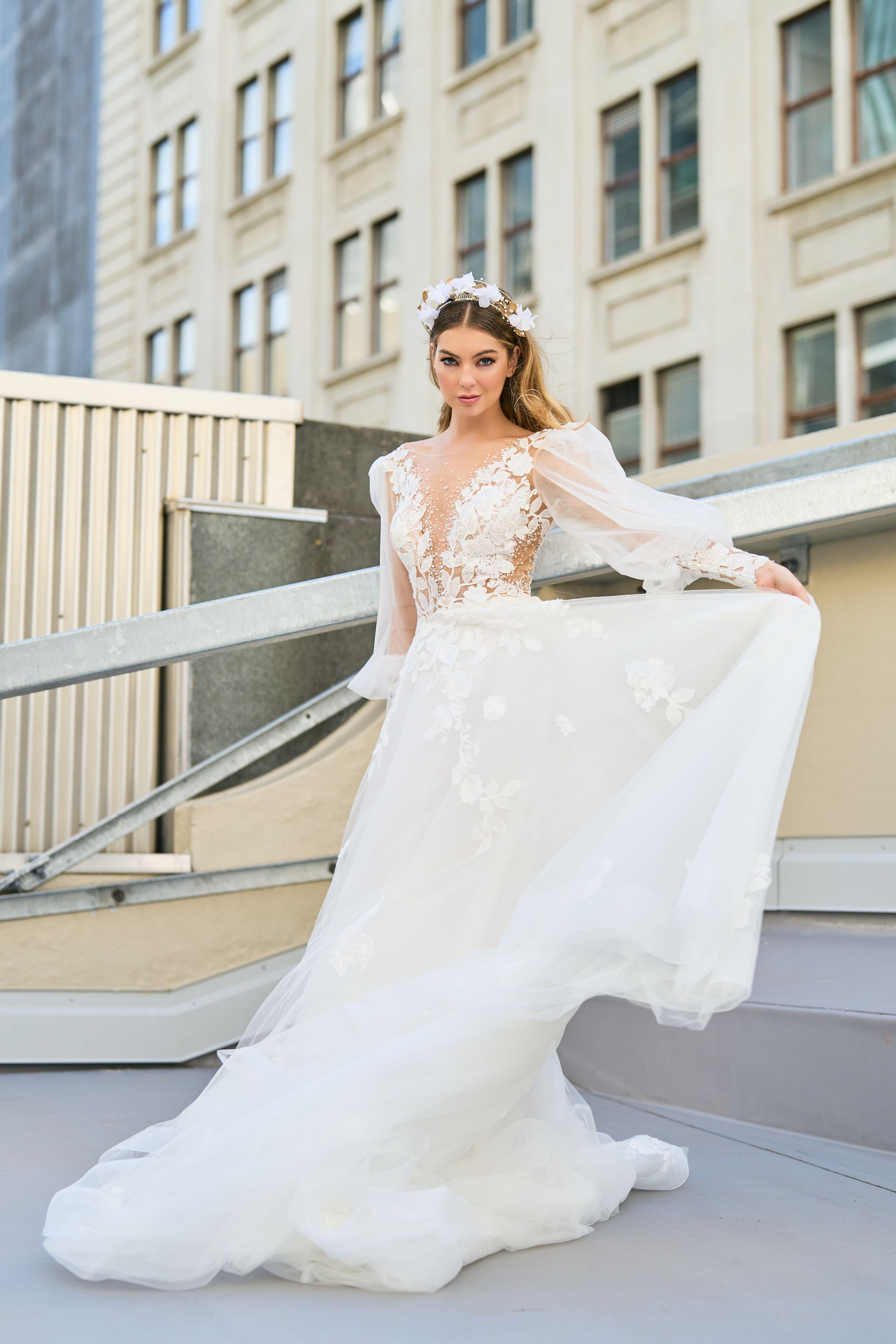A stunning photograph features a young woman posing gracefully on a rooftop terrace, possibly in New York City, with the backdrop of a tan, window-adorned building. The model, who is either Caucasian or Latino, dons an elegant, intricately lacy white wedding dress with a torso adorned in transparent fabric and floral embellishments. Her long, thin sleeves contribute to the ethereal quality of the ensemble. She wears a tiara-like headband of white flowers, with additional petals adorning her head, enhancing her bridal appearance. The model is holding a section of her dress with her left hand, creating a wavy, triangle shape, while her right hand rests subtly behind her back. Her expression is neutral as she gazes directly into the camera, and the cityscape background is softly blurred, placing full emphasis on her and her exquisite attire.